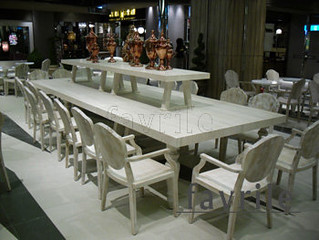The image portrays a banquet-style dining table set within an upscale furniture store or restaurant, characterized by stylish décor and dark walls. The expansive white table, possibly crafted from white marble, has a unique elevated centerpiece—another table with short legs—placed in the middle. This smaller table supports several copper or bronze objects resembling urns or trophies, numbering between five to eight. Surrounding the main table are numerous white wooden chairs, totaling around sixteen: two at each end and seven to eight along each longer side. The chairs appear relatively small and offer minimal support. Additional table and seating displays can be seen scattered throughout the venue, enhancing the overall sophisticated ambiance. The space is well-lit, contributing to its elegant and refined atmosphere.